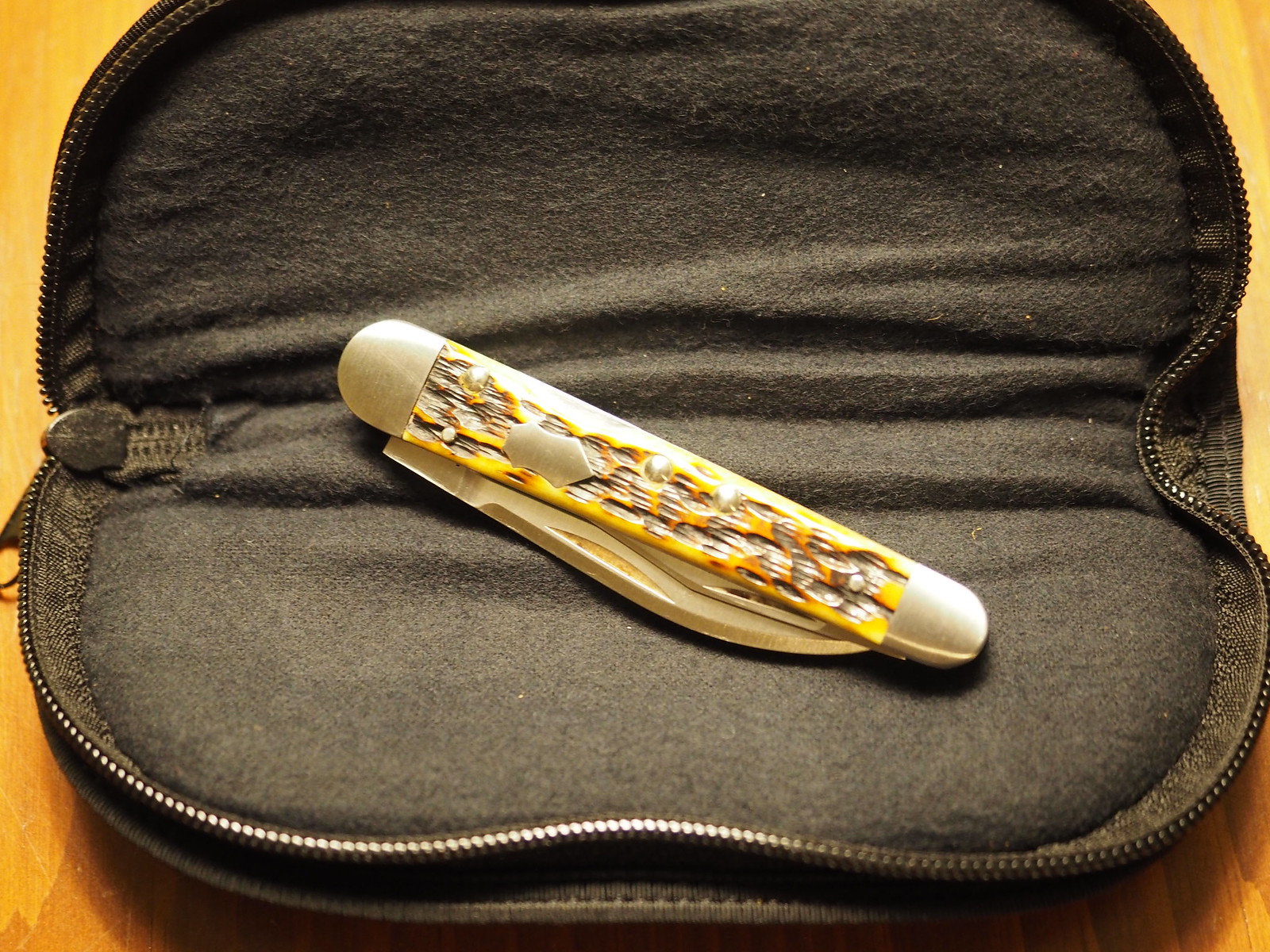The image depicts a pocket knife resting on an open black carrying case, situated on a wooden surface. The case, resembling a padded glasses case with a zipper running around it, has a soft black felt interior. The pocket knife features a bone handle that is predominantly yellow and dark brown, with silver caps on both ends. The handle is detailed with a design and has two prominent screws in the middle, securing the structure, along with smaller screws at the top and bottom. The knife, folded in on itself with highly reflective stainless steel parts, also includes an engraved area on the handle, which is plain. The lighting in the image is from an interior source with a warm yellowish tone, highlighting the knife's metal surfaces.